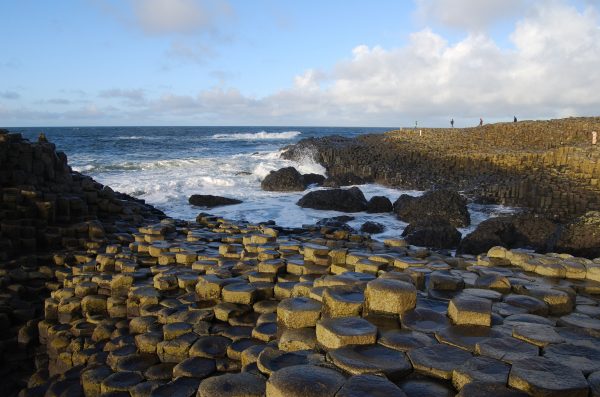This daytime photo, reminiscent of the Devil’s Postpile, captures a striking coastal scene with an inlet leading into the open ocean. The foreground features a fascinating display of volcanic stones, their flat, octagonal tops fitting snugly together like posts emerging from the ground. Some of these stones rise higher than others, creating a varied texture across the landscape. Amidst these stones, which are predominantly gray and brown, are smoother, rounder rocks stacked on top of each other. The ocean in the background displays dark blue waters with white waves breaking towards the shore. At both sides of the inlet are steep cliffs, the right one topped with a light green ridge shadowed at the bottom, where a couple of people can be seen in the distance. Above, the light blue sky transitions to fuller white and gray clouds mostly gathered on the right side. The overall color palette includes shades of blue, gray, black, white, and occasional hints of yellow from sunlight. This semi-professional photo expertly blends the intricate details of the rocks in the foreground with the expansive beauty of the ocean and sky beyond.